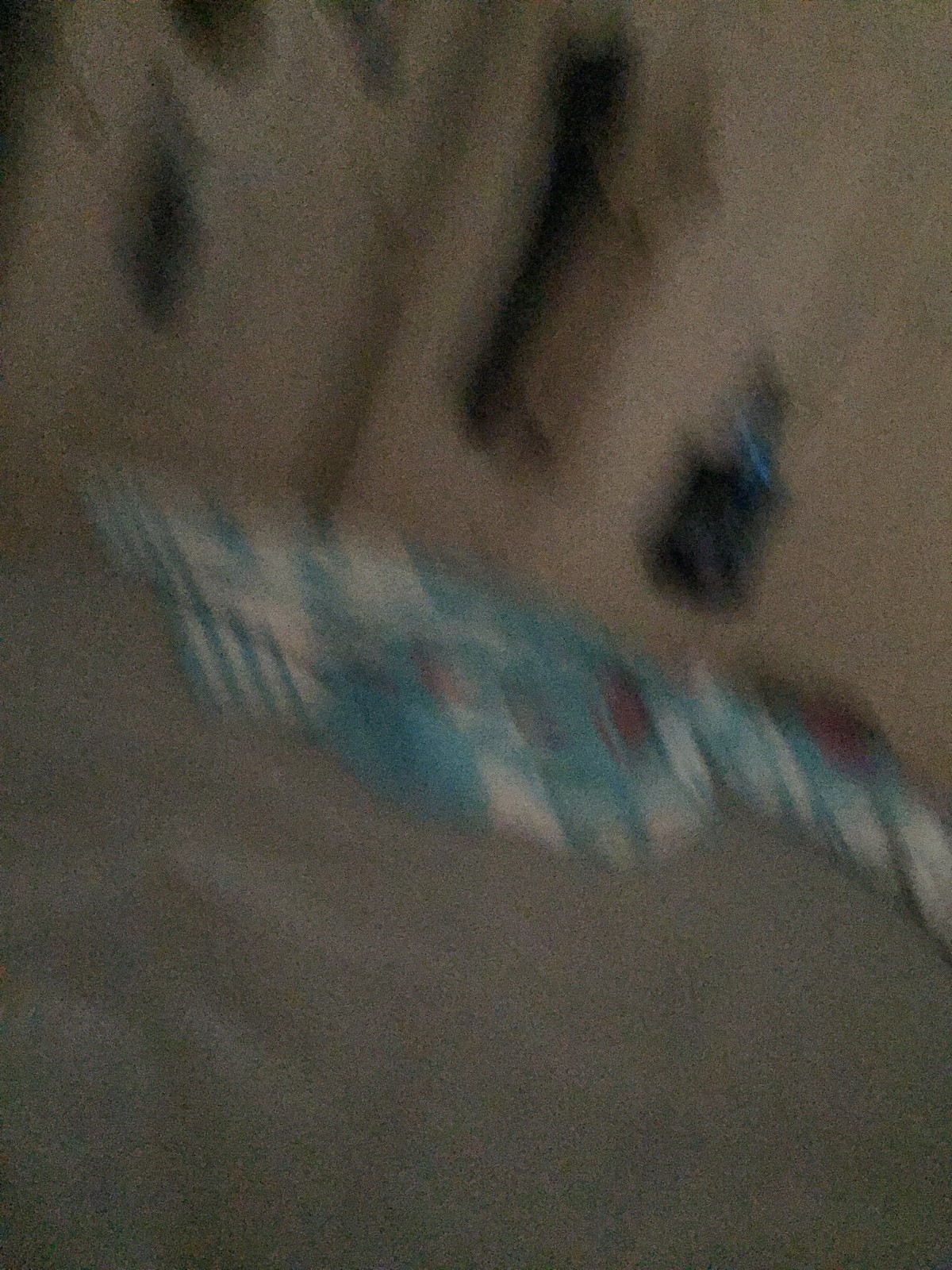This is an extremely blurry photograph, making it difficult to discern distinct details. Dominating the center of the image, there is a blue and white striped object, which also features some red circles—it resembles a blob due to the distortion and could be lying on a flat surface like a gray sheet or possibly a couch. The image appears to be taken at a diagonal angle, with objects sloping towards the right. In the background, there is a structure that seems to be a door frame, above which are hanging some indistinct items. Among these, a black bag is noticeable, along with a blue bag and a tan or creamy-colored item, both casting shadows. The photograph is grainy, with potentially inaccurate colors due to the heavy blur, but additional blurry black objects are visible, contributing to the overall indistinct and fuzzy nature of the image.